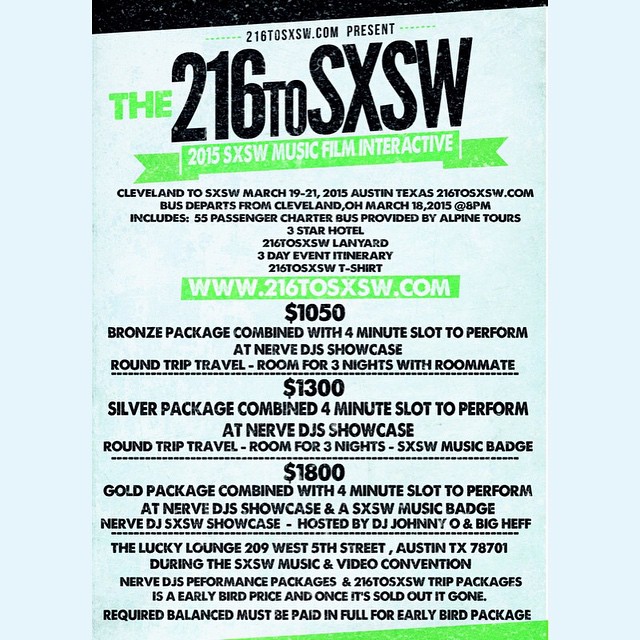The image depicts a detailed promotional poster for the 216-2SXSW 2015 Music, Film, and Interactive Festival. The white poster, adorned with black and green lettering, stands out against a white wall. It announces the "216-2SXSW", an event aimed at connecting Cleveland with the SXSW festival in Austin, taking place from March 19th to 21st, 2015. The poster highlights that three different travel and accommodation packages are available: the Bronze package for $1,050, which includes a 4-minute performance slot, the Silver package for $1,300, and the Gold package for $1,800. All packages offer round-trip travel and room accommodations for three nights with a roommate. Additionally, the address for the event is provided as the Lucky Lounge, located at 209 West 5th Street, Austin, Texas. The website www.216toSXSW.com is cited for further details.